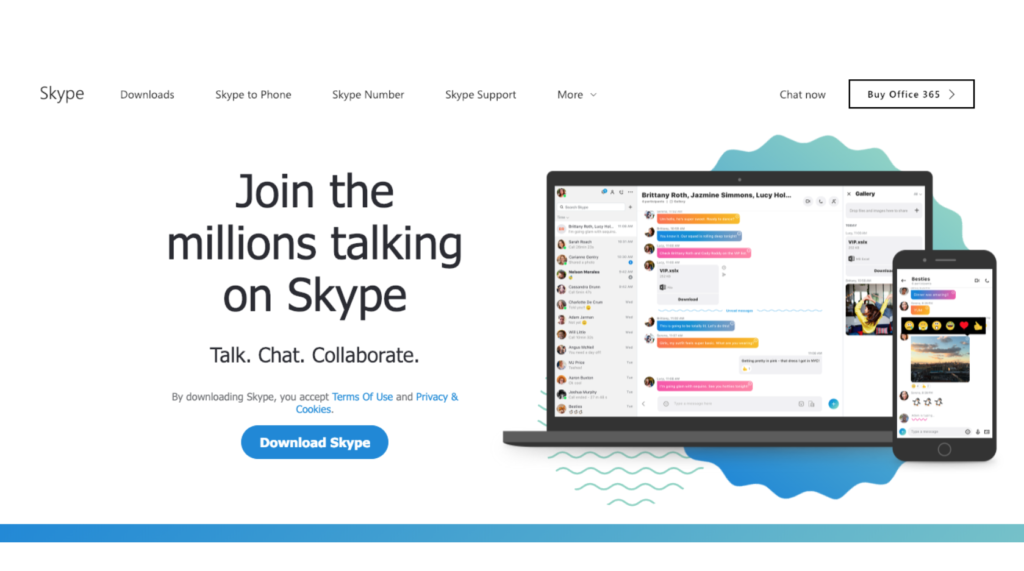This is a screenshot of the Skype website. In the top left corner, the "Skype" logo is displayed prominently in gray lettering typical of the brand. Directly beneath it, there is a menu in smaller gray font listing options: "Downloads," "Skype to Phone," "Skype Numbers," "Skype Support," and "More." Adjacent to "More" is a downward-facing arrowhead indicating a drop-down menu. 

To the right of the menu, "Chat Now" is clearly displayed, followed by a black-outlined rectangle containing the text "Buy Office 365" and a right-pointing arrowhead.

Centered on the page but slightly offset to the left, the message "Join the Millions Talking on Skype" is boldly written in large black text. Directly below it, in smaller black letters, are the words "Talk. Chat. Collaborate." Following this, in even smaller text, the disclaimer reads, "By downloading Skype, you accept Terms of Use and Privacy and Cookies," with "Terms of Use" and "Privacy and Cookies" highlighted in blue to indicate clickable links.

Beneath the text, a dark blue, elongated oval button stands out with the words "Download Skype" in white, inviting users to click and start the download process.

Towards the right side of the screen, a black laptop displays the Skype application, emphasized by its vibrant screen. In front of the laptop, a black smartphone also running Skype is shown, with an active conversation visible on its screen. A strip of emojis is displayed towards the middle but slightly towards the top of this section, adding a playful element.

The background features an artistic design of a squiggly circle pattern transitioning from an aqua green color at the top to blue at the bottom. To the left, several wave symbols enhance the visual appeal of the page.